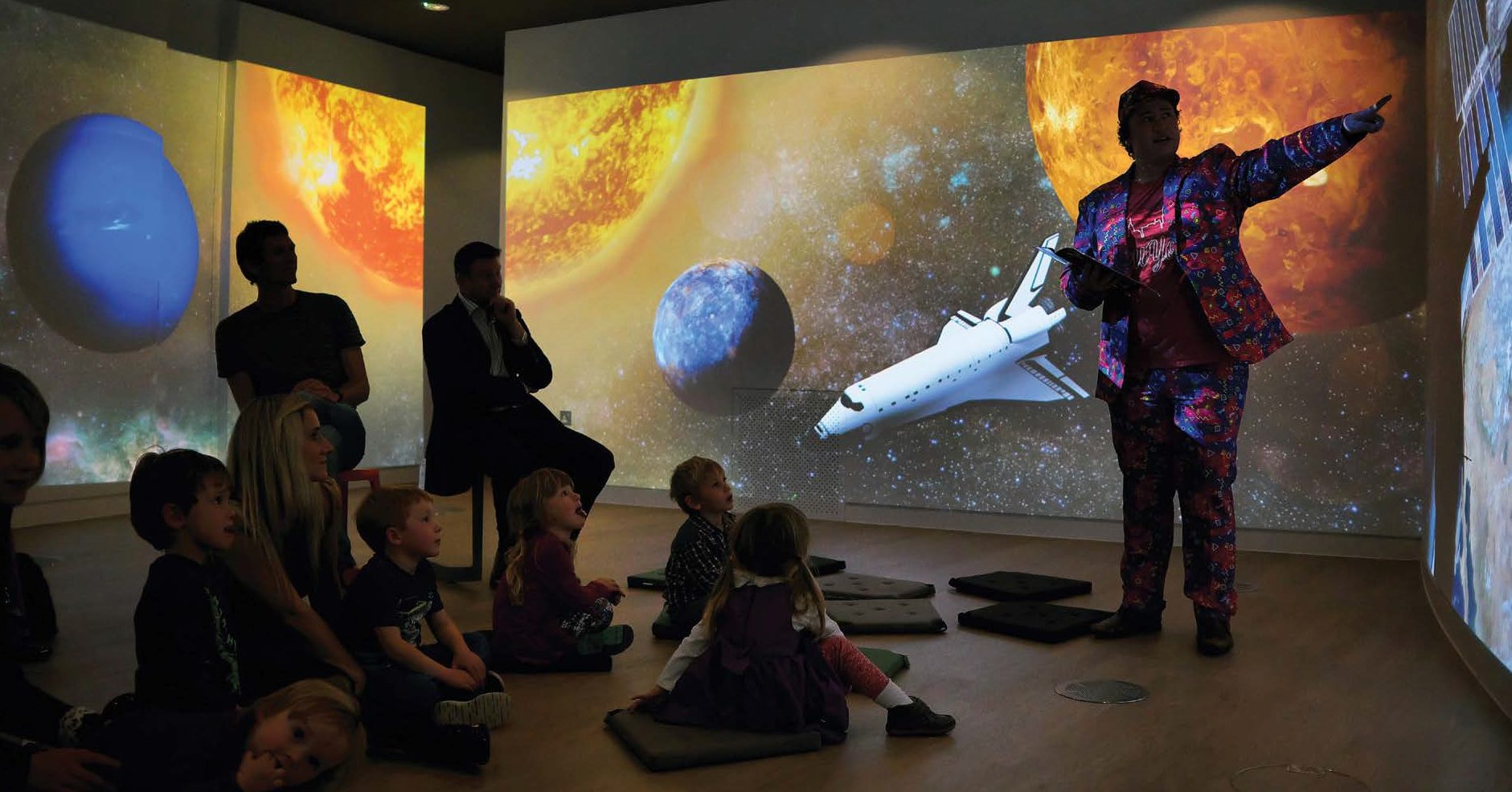The photograph captures an indoor scene illuminated by artificial lighting, where a scientific lecture about space is taking place. The image, horizontally rectangular in shape, presents no discernible border. The setting appears to be a museum adorned with vividly painted walls that feature celestial imagery, including a large yellow sun, various planets in shades of blue, red, orange, and brown, and a white space shuttle. The walls create an immersive environment, resembling a star-speckled space background.

In the bottom center of the image, a group of young children sits attentively on small gray mats placed on a light wood laminate floor. The kids, some sitting cross-legged, are entranced by the lecturer. The speaker, likely a man, stands on the far right side of the frame, engaging the audience by pointing at a projector screen. The screen's light casts an illuminated glow over his colorful attire, which includes a blue suit with red tie-dye patterns and a baseball cap. He holds a tablet or book in one hand as he directs the children's attention to the projected material.

To the left of the children, a few adults are seated on chairs, partially obscured in the shade, attentively observing the presentation. There's also an adult among the children on the floor. Overall, the photograph encapsulates an educational and visually stimulating environment, enriched with space-themed decorations and a dynamic presentation that captivates its young audience.